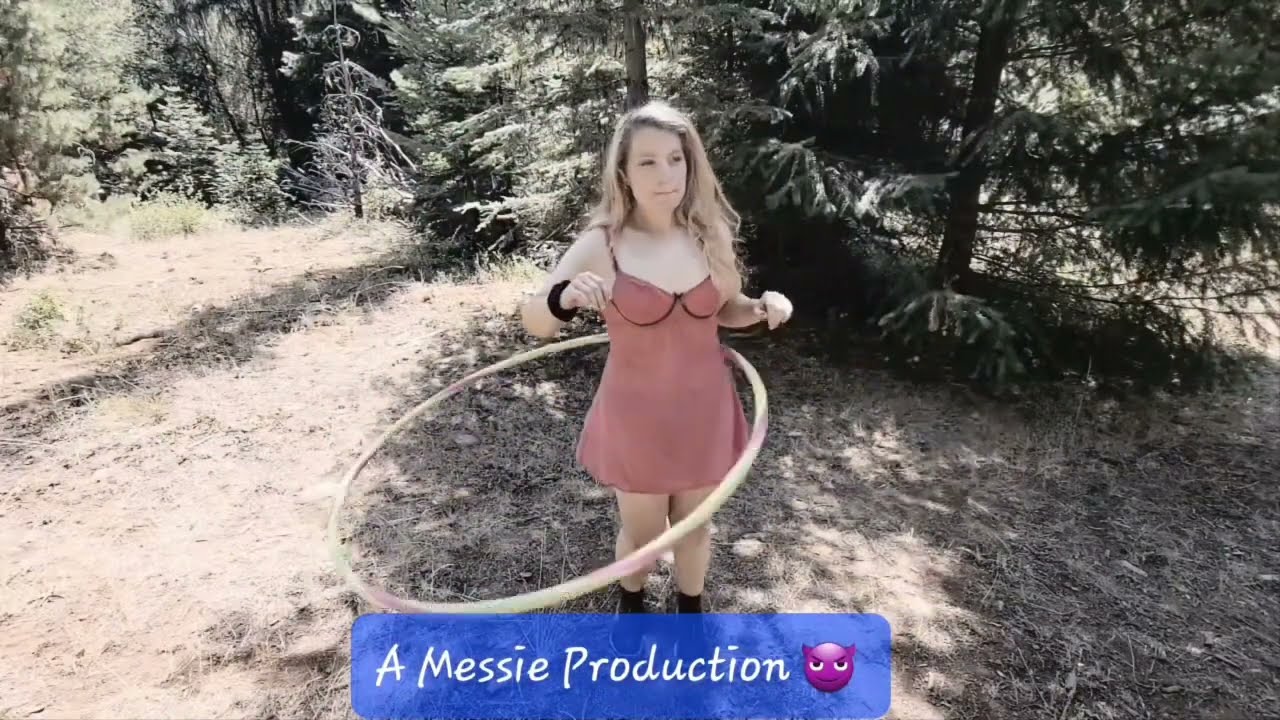The image depicts a Caucasian woman standing amidst a forest of tall, green pine trees, engrossed in hula hooping. She has long blonde hair parted to the side and wears a thigh-length, dark salmon pink camisole dress with spaghetti straps. Her right wrist is adorned with a black scrunchie. The woman is seen with her elbows fixed to her side, concentrating on maintaining the rhythm of the hula hoop, which is rainbow-colored and spins around her waist. She sports black socks and possibly black shoes, though they are obscured by a transparent blue banner located at the bottom center of the image. This banner, beveled in white, reads "a Messi Production," with "Messi" spelled as "M-E-S-S-I-E" and is complemented by a smiling purple devil emoji. The photograph, taken outdoors during the daytime, features a sparse forest floor, adding to the wilderness ambiance. The woman is looking slightly to her right, her mouth closed in concentration as she engages with her activity, surrounded by the natural, serene environment.